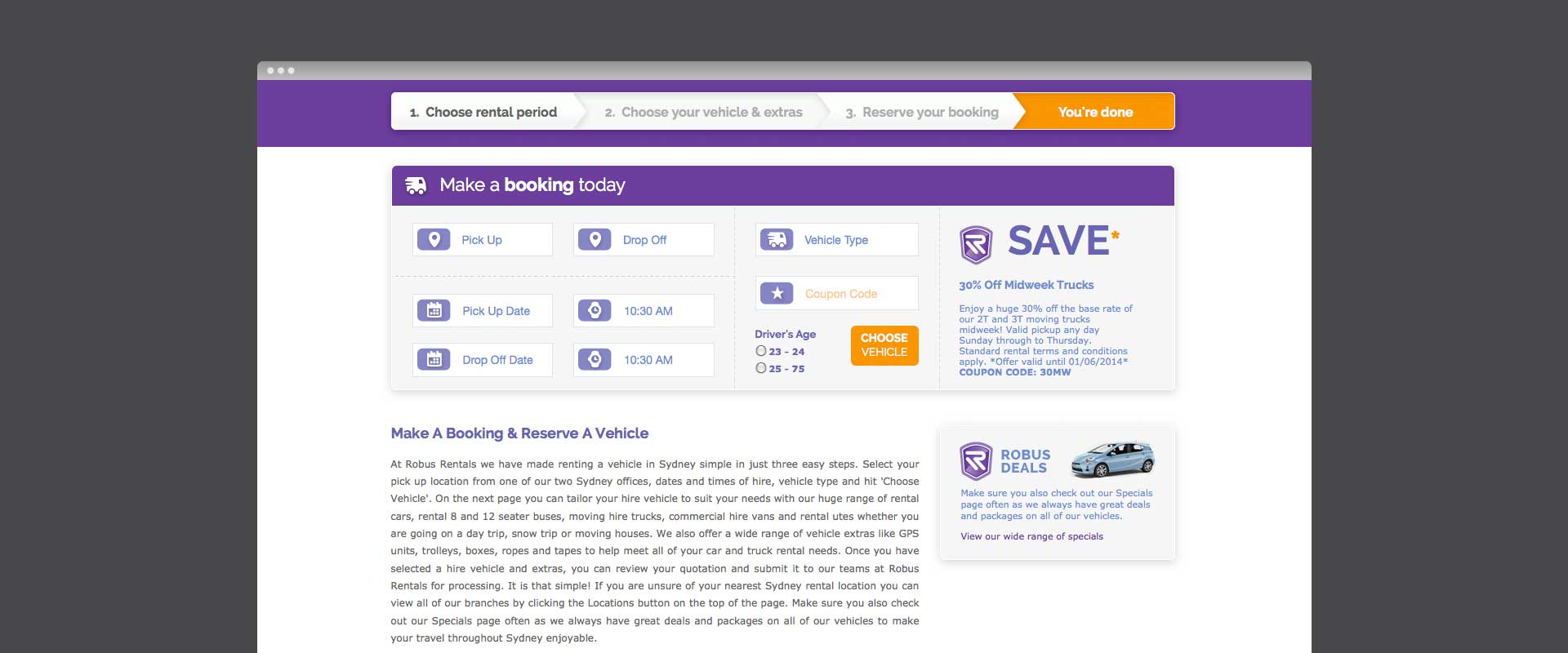This screenshot captures a desktop environment that appears to be running on a Mac, as indicated by the signature three colored dots (red, yellow, green) located at the top-left corner. Spanning the screen right below these dots is a horizontal purple strip. This image appears to be from a vehicle rental website, organized into a three-step booking process.

At the top of the interface, Step 1 is prominently highlighted in black text on a white background, reading "Choose rental period." Following this, Step 2, which is displayed in light grey text on white, reads "Choose your vehicle and extras." Finally, Step 3 is titled "Reserve your booking." Completing the steps, an orange tab on the right side, with white text, confidently declares "You're done."

Directly below the step indicators, a detail section on a white backdrop features a short purple strip containing an icon of a small truck or van, accompanied by a prompt in white text encouraging users to "Make a booking today."

Further down, various selection options are provided to customize the rental experience. Users can specify their "Pick-up" and "Drop-off" locations, as well as the "Vehicle type." The "Pick-up date" field remains unset, but the "Pick-up time" is preset to 10:30 AM. Likewise, the "Drop-off" information mirrors these details, with an unset date and a time of 10:30 AM. 

There is also an appreciable dropdown for selecting the driver's age range, offering categories such as "23-24" and "25-75," with a subtle implication that drivers aged 23-24 might be subject to additional scrutiny or conditions. The user is also prompted to choose the type of vehicle required for their booking.

Overall, the layout is methodical, presenting a clear flow from initial selection to final reservation, aiming to streamline the vehicle rental process for the user.